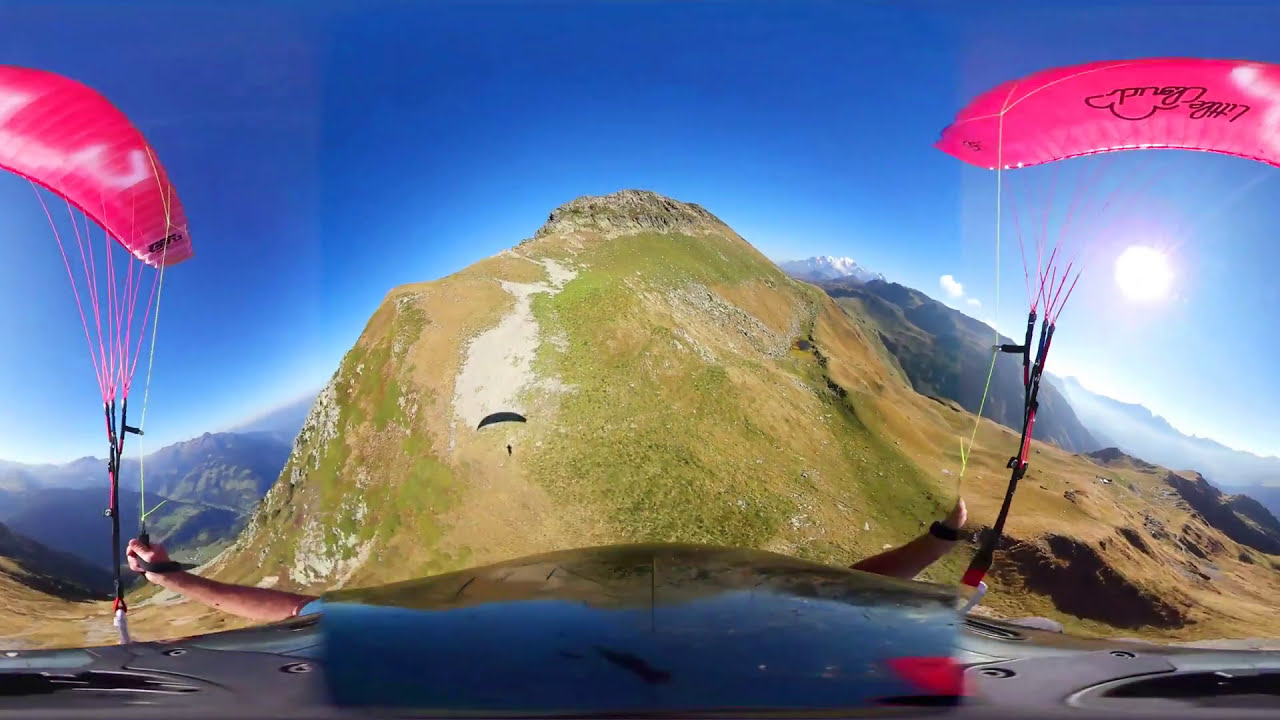The image captures the exhilarating moment of a paraglider in flight, viewed from a fisheye lens likely mounted on his helmet, offering a wide 360-degree perspective. Set against a striking mountainous backdrop, the scene unfolds during late evening, as evidenced by the low-hanging sun on the right side of the frame. The sky above is a clear expanse of blue, punctuated by distant clouds nestled between the rugged peaks. The central focus is a massive hill or mountaintop that dominates the middle of the image. The paraglider, a Caucasian male, extends his arms as he maneuvers the vibrant pink parachute that stretches across both the left and right sides of the frame, reflecting the wide-angle view. Multiple other parachutes dot the sky, positioned to the left and right of the central peak, adding a dynamic element to the serene yet adventurous landscape. The range of colors—blue, white, yellow, pink, brown, tan, and black—enhances the visual depth, portraying a vivid and detailed outdoor setting in the heart of nature's grandeur.